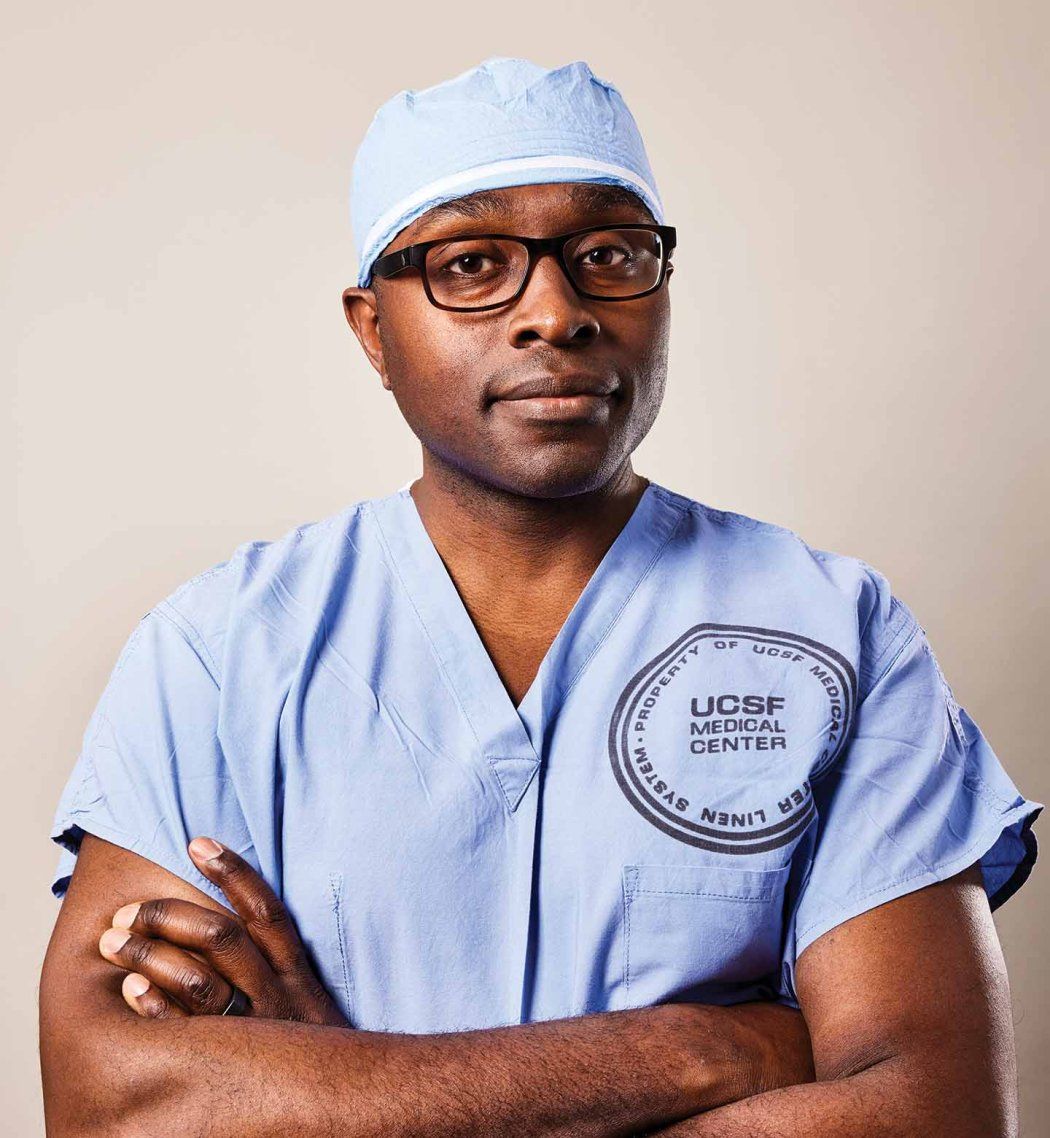This is a detailed image of an African-American male medical professional, likely a surgeon, dressed in blue scrubs and a matching blue scrub cap with a white stripe at the base. His scrubs prominently display the words "Property of UCSF Medical Center" enclosed in a circle on the chest area. The man is facing the camera, situated front and center, with a clear background ensuring all focus is on him. He is wearing black glasses, a black wedding ring on his left hand, and is well-shaven with no visible hair. His arms are crossed, and he projects a serious, yet mildly challenging expression, as if saying, "try me." He exudes confidence and professionalism, captured in a pose that reveals his dedication to his vocation. The image lacks any additional text or distractions, making the man and his attire the focal points.